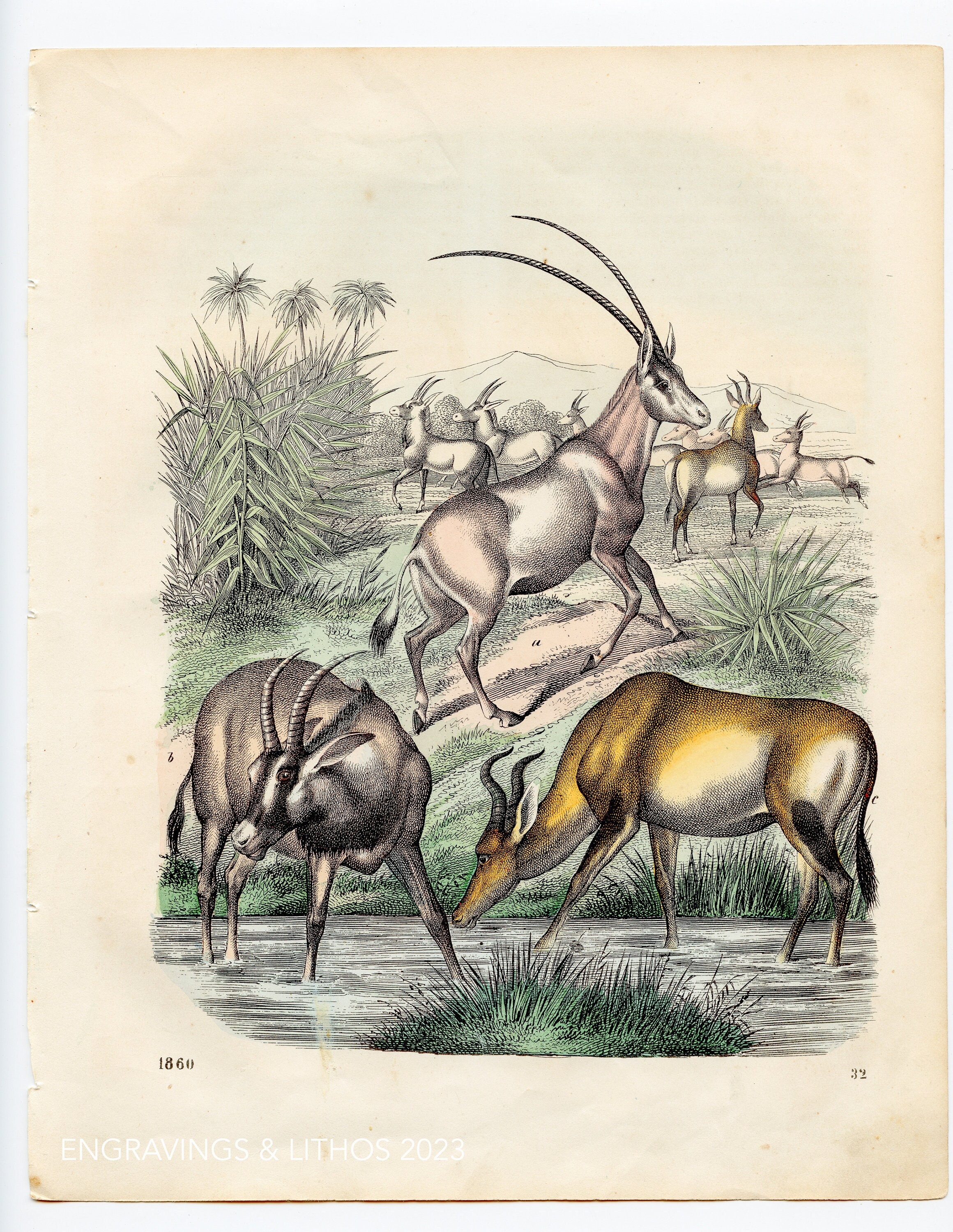This detailed illustration captures a serene scene of antelopes and gazelles at a watering hole. In the foreground, a brown gazelle with horns crouches down while another gazelle, positioned to its left, stands gazing into the distance. Both animals appear alert, with the crouching gazelle seemingly glancing at its companion. Nearby, an antelope stands ankle-deep in the water, drinking, while another with impressive, elongated horns climbs a nearby mound of dirt. This antelope has a striking purplish-brown hue, contrasting with the lighter brown and golden tones of the other animals. The watering hole is surrounded by lush, vibrant greenery and tall, spiky plants with shaggy flowers. In the background, more gazelles and antelopes are visible, adding depth to the scene. A mountain range looms in the distance under the daylight sky, completing this 1860 dated artwork.